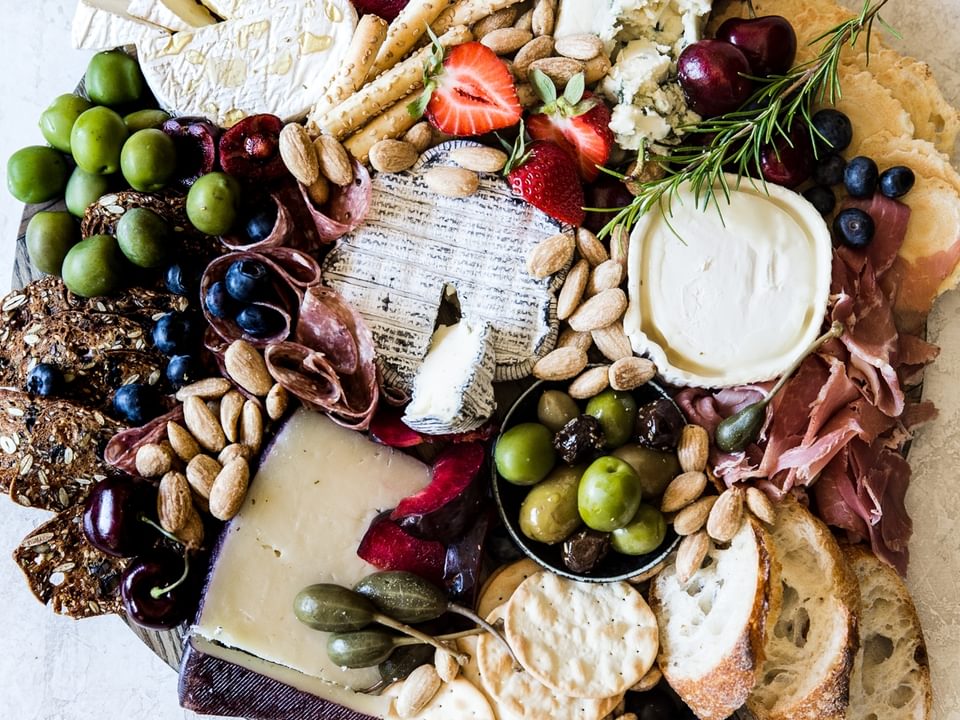This top-down, color photograph shows a beautifully designed charcuterie board, meticulously arranged and bursting with a variety of delectable snacks. The board features an array of meats, cheeses, breads, crackers, nuts, fruits, and dips, creating a visually appealing and mouth-watering spread. Among the meats are slices of prosciutto and salami, their reddish hues contrasting with the white and pale-yellow cheeses, which range from soft to hard, possibly including varieties like blue cheese, parmesan, and Gruyere.

The breads are diverse, featuring both light sourdough and darker breads such as pumpernickel, alongside an assortment of white and flat crackers, some of which are long, stick-like with sesame seeds. Scattered throughout the board are green and black olives, almonds, and fresh herbs like rosemary. Bright red strawberries, deep red cherries, and a handful of blueberries add a splash of vibrant color, enhancing the overall aesthetic. The board also includes potential dips or soft cheeses, perfect for pairing with the other elements on this enticing charcuterie display.